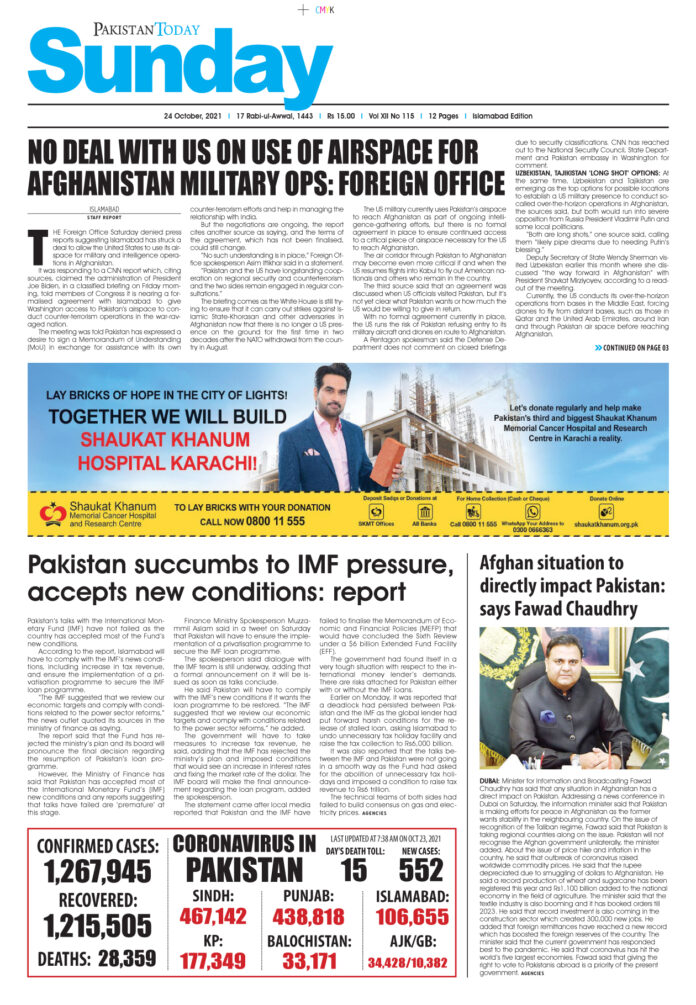This image features the front page of the October 24, 2021, Sunday edition of Pakistan Today, presented in a traditional broadsheet format. 

In the upper left corner, the masthead "Pakistan Today" is prominently displayed, with "Pakistan" in black and "Today" in light blue. Above this, the word "Sunday" is large and bold in light blue, indicating the special weekend edition. A couple of black lines separate these elements, and beneath them, the date "24 October, 2021" is listed, along with the note that this is an "International Edition" with "12 pages." The volume number is also specified.

The main headline, left-justified in large, bold black font, reads: "No deal with U.S. on use of aerospace for Afghanistan military ops: Foreign Office." Below the headline, the related article spans four columns, though the text is too small to read except for the prominently large initial "T." The article occupies roughly a third of the front page, with the text not continuing beneath the headline. It stops at the same height as the top of the headline and indicates a continuation on another page.

Below the article, a full-width, full-color advertisement appeals to the viewer. The ad features a man with dark hair and a mustache, dressed in a medium blue sports jacket and an open-neck pink shirt. He holds a brick in his left hand. To his right (the left side of the page from the viewer's perspective), the tagline "Lay bricks of hope in the city of light. Together we will build." is displayed in black, with "Shawkat Khanum Hospital Karachi!" in red. Additional text to the right of the figure includes contact information, suggesting viewers call now to donate.

Beneath the advertisement are two more articles. The one on the left occupies three columns with the headline: "Pakistan succumbs to IMF pressure, accepts new conditions: Report." Adjacent, on the right, is a one-column article titled: "Afghan situation to directly impact Pakistan: says Fawad Chaudhry." Accompanying this article is a rectangular image of Fawad Chaudhry, sitting at a desk, dressed in a black shirt with a Pakistani flag prominently visible in the background.

In the lower left corner, a graphic details the confirmed coronavirus cases in Pakistan, breaking down the numbers by region, including Punjab and Islamabad. The total confirmed cases listed exceed one million, with precise figures provided.

This comprehensive layout highlights the newspaper's focus on key national and international issues, supported by visual and textual elements that enhance information delivery.